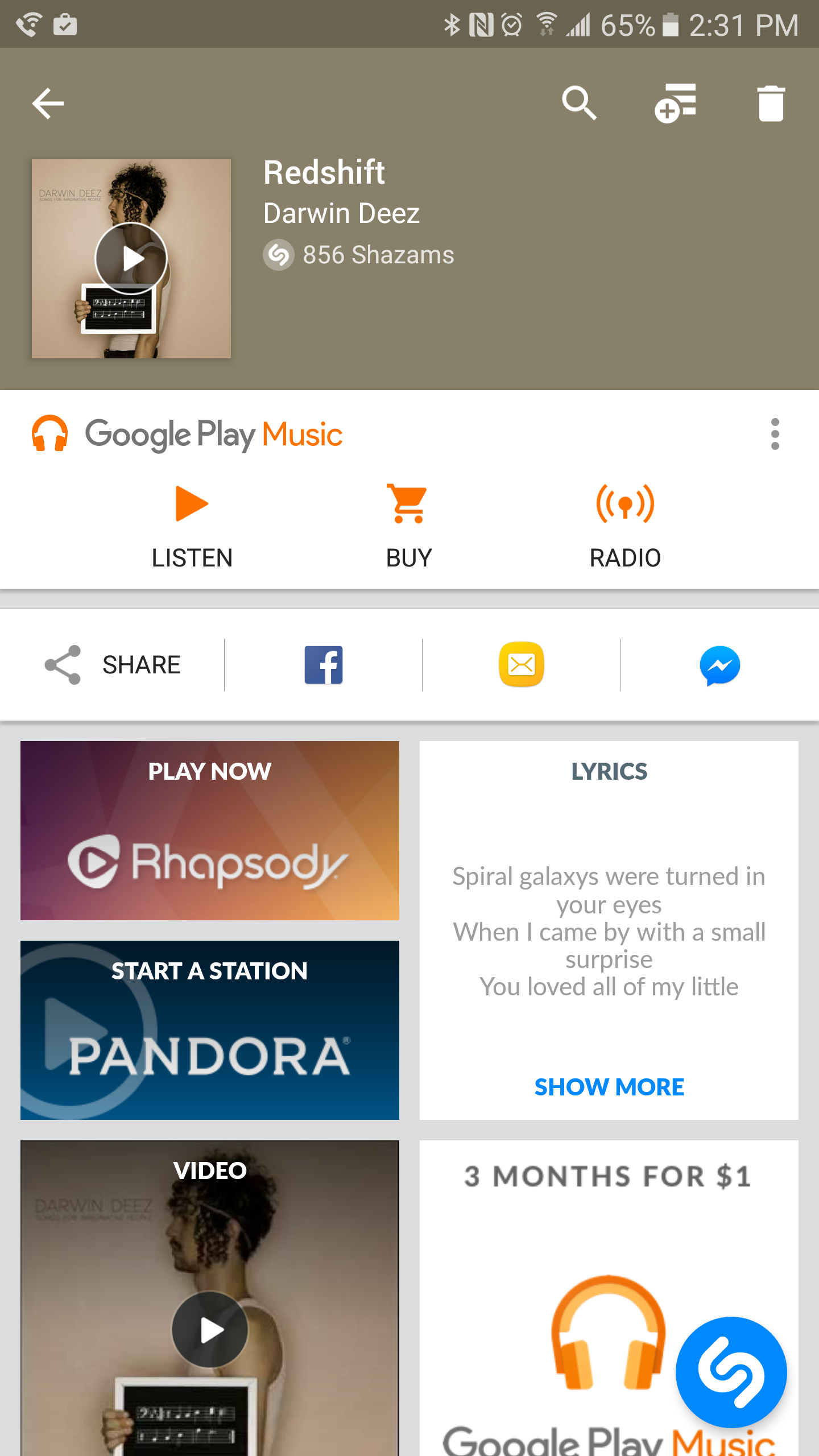The image displays a tablet screen opened to the Google Play Music app. At the top of the screen, there's a status bar showing the time, date, battery life, and other indicators. Beneath this is a user interface featuring a search magnifying glass icon and a recycle bin section.

Central to the screen is a playing media section where a song titled "Redshift" by Darwin Dees is highlighted. The interface shows options for listening by radio and sharing via Facebook, email, and Messenger. Below this section, there's an option to view the song's lyrics and a promotional banner offering three months of Google Play Music for one dollar.

Additionally, there is a "Play Now" button for another song titled "Rhapsody." Further down, a "Starter Station" option is available, suggesting that users can start a music station, potentially through a membership with Pandora.

The screen also features a thumbnail image of "Redshift" by Darwin Dees at the bottom, mirroring the main song display at the top but without visible text, only an option to play or select the song. The overall layout is indicative of a user-friendly music streaming interface designed to streamline music discovery and playback options.